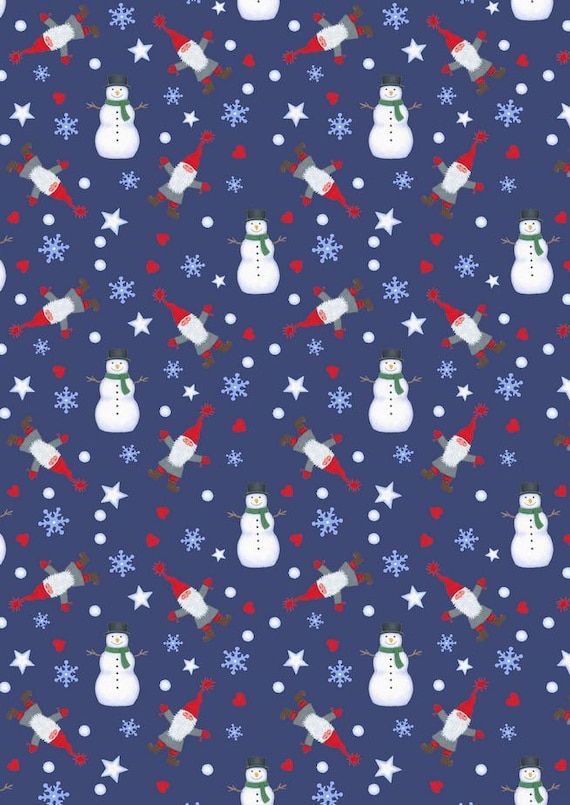The image depicts a piece of Christmas-themed wrapping paper with a dark blue background, adorned with a repeating pattern. The primary elements are frosted snowmen and playful gnomes, positioned in various orientations as if frolicking in the snow. Each snowman, designed in a classic cartoon style, features a black top hat, a carrot nose, stick arms, a green scarf, and five coal buttons. Surrounding the snowmen are gnomes, each with a long white beard, a pointy red hat topped with a pom-pom, white gloves, a red shirt, white socks, and blue shoes. The background is filled with different shapes and sizes of snowflakes, stars, white and red dots, and red hearts, all creating a festive atmosphere. The characters and icons repeat seamlessly, evoking the feel of traditional holiday wrapping paper.